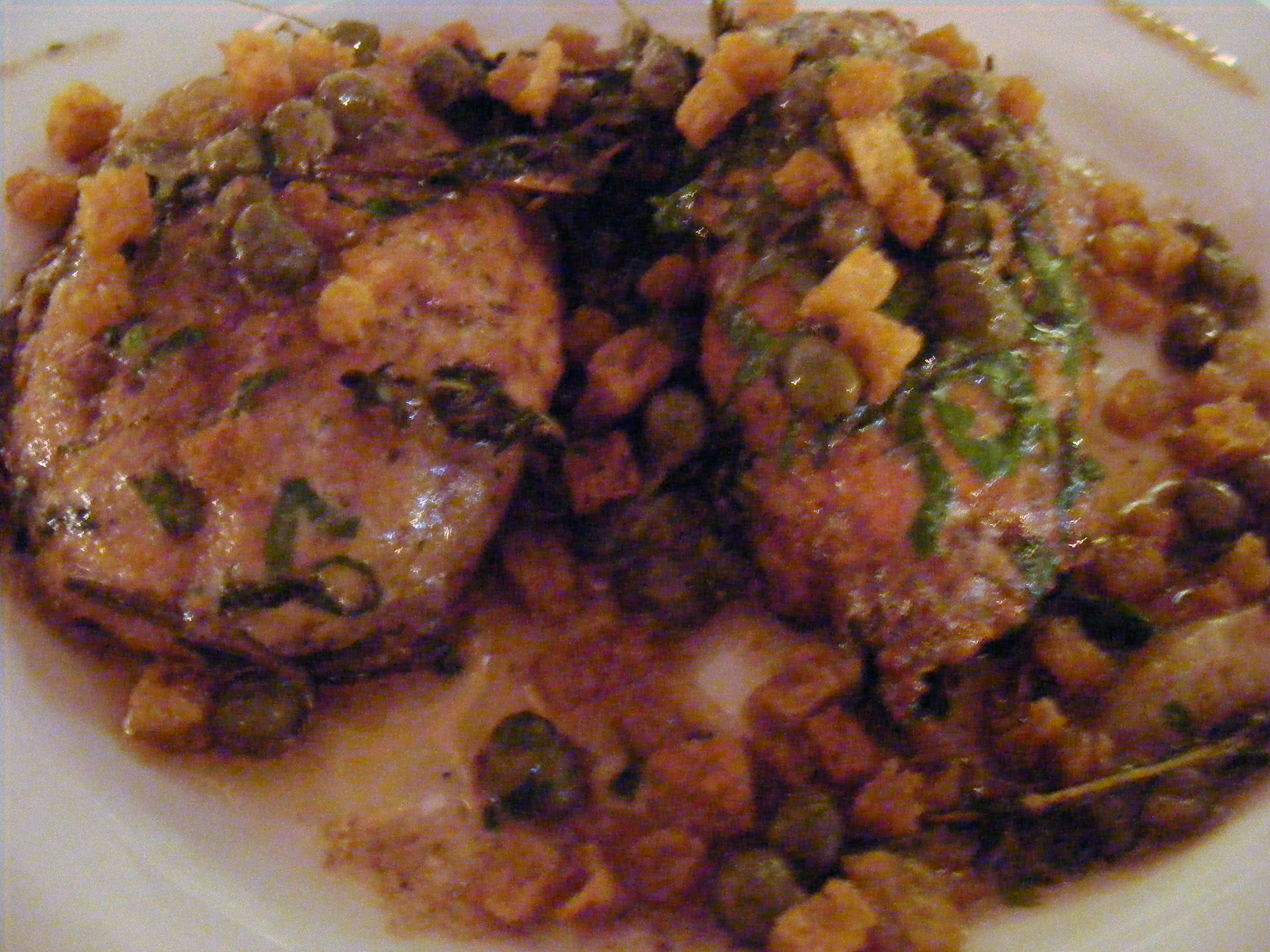The image showcases a close-up of a richly glazed, saucy meal centered on a white plate. Dominating the dish are two large, orange-brown chicken breasts, positioned centrally. These are generously topped and surrounded by a vibrant mix of vegetables: bright yellow corn, green peas or chickpeas, and various green leafy herbs. Additional colorful elements, including green olives and possibly lentils, can be seen scattered around, contributing to the dish's overall visual appeal. The plate itself features subtle gold accents at the edges. The food arrangement is dense, with vegetables nestled between and around the chicken, creating a visually engaging and appetizing display. The surface is shiny and greasy, indicating a rich, succulent preparation.